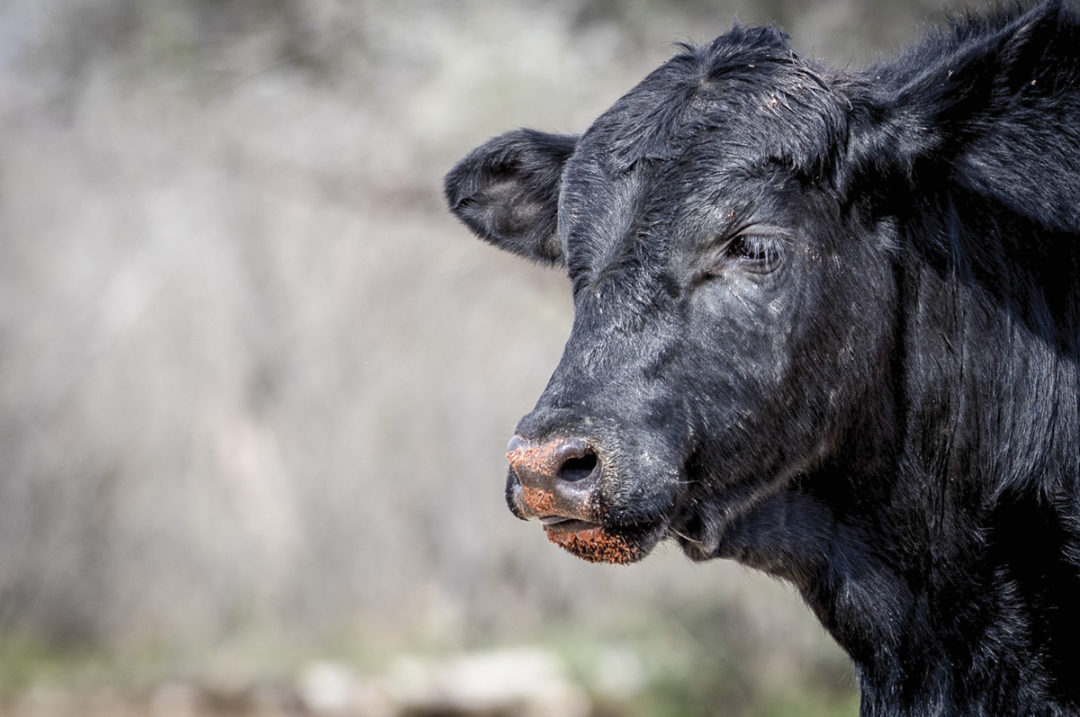Captured outdoors during a time that is likely from spring to early fall, this photograph showcases a primarily black cow, positioned towards the right-center of the frame and angled slightly towards the viewer. The background is heavily blurred, appearing gray with only a hint of green on the ground, suggesting foliage that is out of focus. The cow, which might be an Angus breed, is facing left with its head slightly down. Its dark black fur is highlighted by a small area of pinkish-red on its snout, possibly indicating contact with red dust or grain. The cow's ears stick out noticeably; one appears to stand up straighter than the other. The animal's expression looks serious, with the eyes partially closed or appearing narrow. The cow's distinctive cowlick is visible on the top of its head. Even though there's some debate whether this animal might be a bull or a cow, the absence of horns hints towards it being a female.